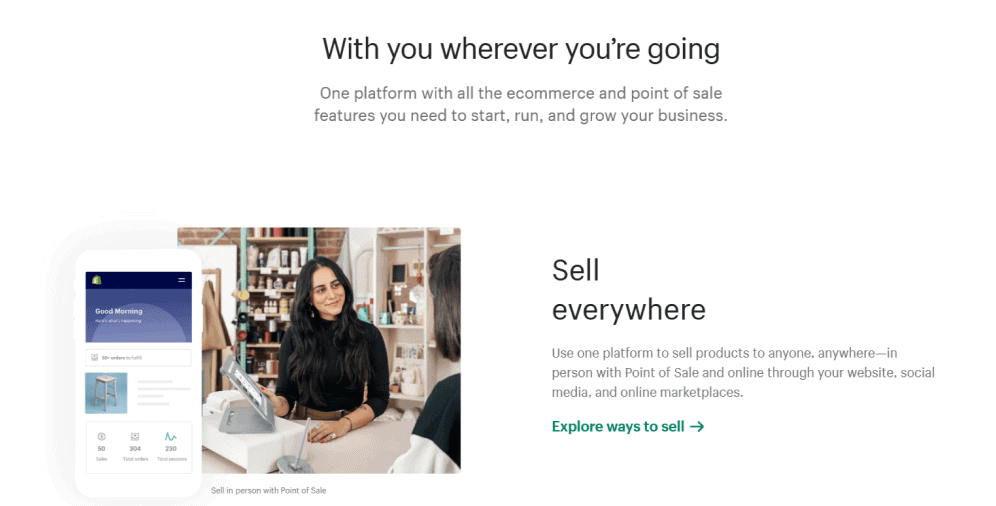The screenshot displays a section of a website designed for e-commerce and point-of-sale solutions on a white background. At the very top, black text reads: "With you wherever you're going." Below this, another line of text states: "One platform with all the e-commerce and point-of-sale features you need to start, run, and grow your business."

The middle section of the screenshot features a photograph on the left side. It depicts a female standing behind a counter, likely in a retail setting. Behind her, shelves filled with various bottles are visible, indicating she may be in a shop that sells drinks or similar items. She holds a tablet, suggesting she may be processing a sale or inventory. Another person appears to be interacting with her from the other side of the counter.

Adjacent to this image, there is a rectangular pop-up box with a gray background that says "Good morning." Below this greeting, there is a small picture of a stool.

On the right side of the screen, text reads: "Sell anywhere. Use one platform to sell products to anyone, anywhere, in person with point of sale, and online through your website, social media, and online marketplaces." Further down, a green text reads: "Explore ways to sell," accompanied by an arrow pointing to the right, inviting users to learn more.